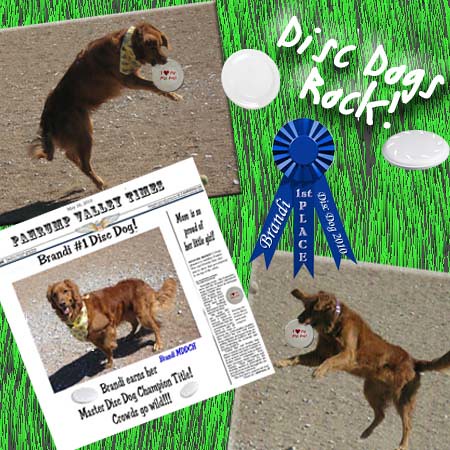The image is a vibrant and detailed collage celebrating Brandy, a brown dog with a bandana, who has achieved the Master Disc Dog Champion title. The entire background is filled with a rich green, resembling a lush grassy field. At the top right, several colorful frisbees are scattered, emphasizing the disc dog theme. Positioned slightly off-center to the right is a prominent dark blue ribbon proclaiming, "Brandy First Place Disc Dog 2010."

In the bottom left corner, there's a slanted newspaper clipping from the Pahrump Valley Times, highlighting Brandy's achievement with the caption, "Brandy earns her Master Disc Dog Champion title. Crowds go wild." Alongside this, to the bottom right, Brandy is captured mid-air, leaping to catch a white disc adorned with red text. This action shot, repeated in the upper left corner, showcases Brandy’s agility and skill.

Overlaying the green grass drawing in white letters is the enthusiastic motto, "Disc Dogs Rock!" beneath which is a symbolic image of a frisbee, underscoring the dynamic sport. The collage, with its rich blend of photographs, text, and drawings, seems lovingly compiled to honor Brandy’s impressive disc dog accomplishments.